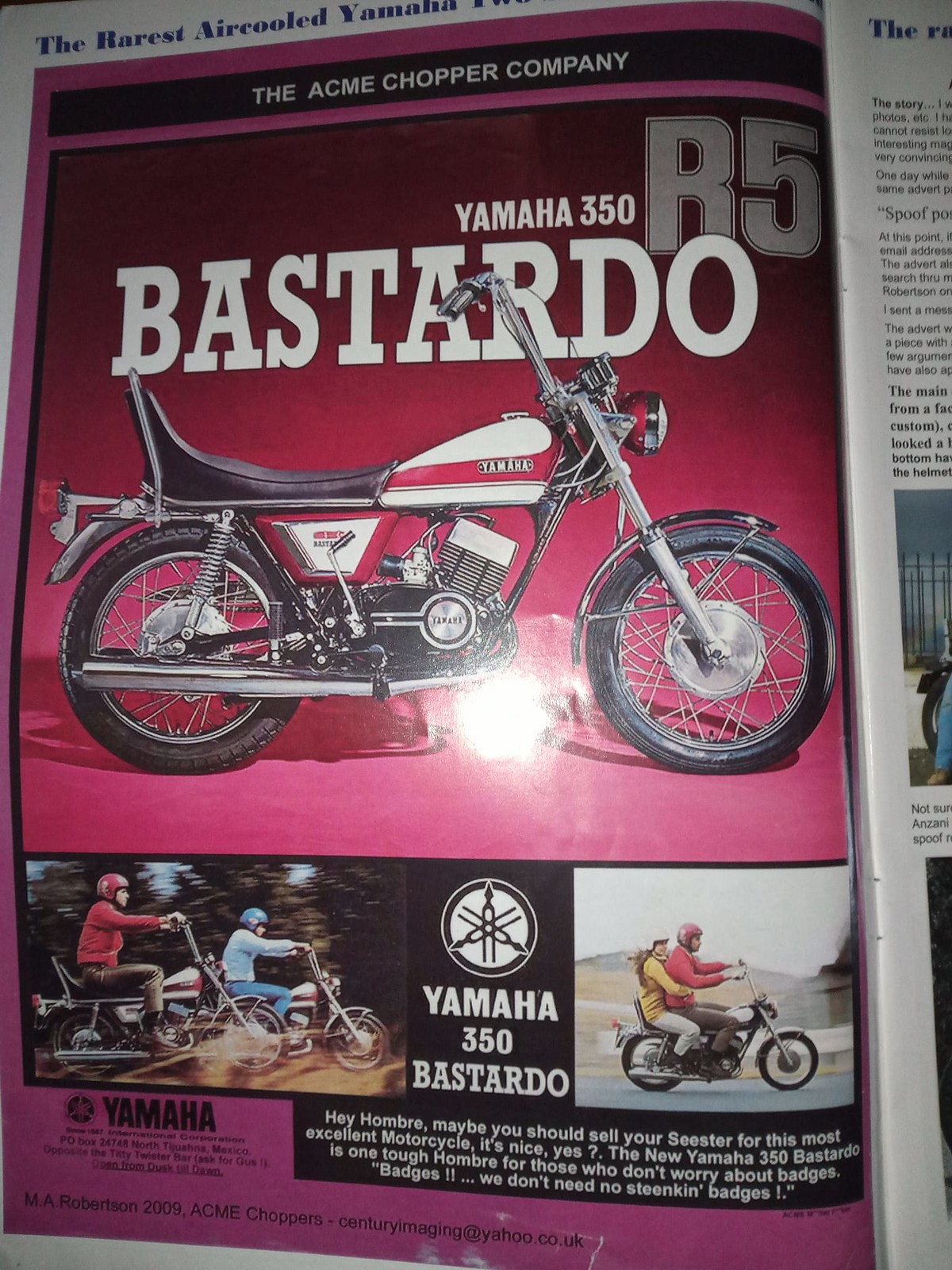This full-color, full-page magazine advertisement features a classic Yamaha 350 R5 Bastardo motorcycle. The ad is set against a rich plum or dark cyan background and prominently displays the title "Acme Chopper Company" at the top. The main image showcases the vintage motorcycle in red, white, and black colors, with striking details such as chrome handlebars and arm, a thin black fender, and a large silver exhaust pipe. The motorcycle, angled to the right, features a white, red-striped tank and a long black seat designed for two riders, curving up at the rear.

Above the motorcycle, the text "Yamaha 350 R5 Bastardo" is written in various font styles and sizes, with 'R5' in a large gray outline and 'Bastardo' in a bold white font. The bottom part of the advertisement includes photos of people riding the Yamaha 350 R5 Bastardo; in one, a person in a red jacket is off-roading through a forested area, and in another, a couple - a woman in a yellow jacket riding as a passenger and a man in a red jacket driving - are navigating a countryside road. The ad humorously states: "Hey hombre, maybe you should sell your sister for this most excellent motorcycle. It's nice, yes? The new Yamaha 350 Bastardo is one tough hombre for those who don't worry about badges. Badges? We don't need no stinking badges."